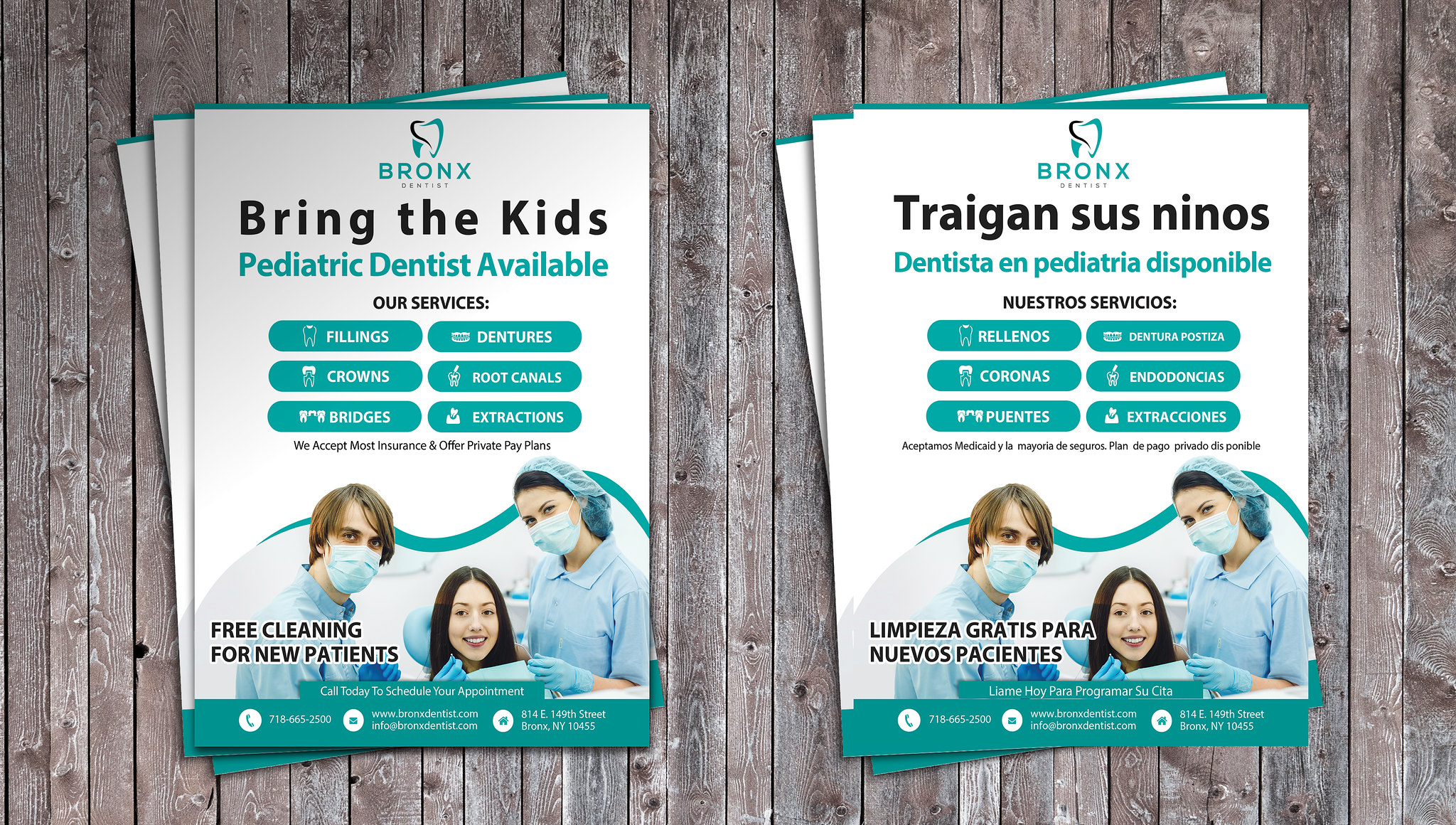The image showcases a digitally-created photo of two identical stacks of pamphlets, positioned side-by-side on a wooden background resembling a picnic table. Each stack contains the same flyer, with the left pile in English and the right in Spanish. The pamphlet header reads "Bronx" followed by the message "Bring the Kids, Pediatric Dental Services Available." Below this, the flyer lists dental services offered, including fillings, crowns, bridges, dentures, root canals, and extractions, along with a note that most insurance plans are accepted and private pay plans are available. At the bottom, a photograph depicts two dental professionals, donned in blue dental attire, hairnets, and face masks, tending to a smiling patient in a chair. The flyer also highlights a special offer of free cleanings for new patients, accompanied by contact details: phone number, URL, email address, and a physical location on 149th Street in the Bronx. The Spanish version retains all design elements, merely translating the text. The overall color scheme of the pamphlets consists predominantly of white and teal.